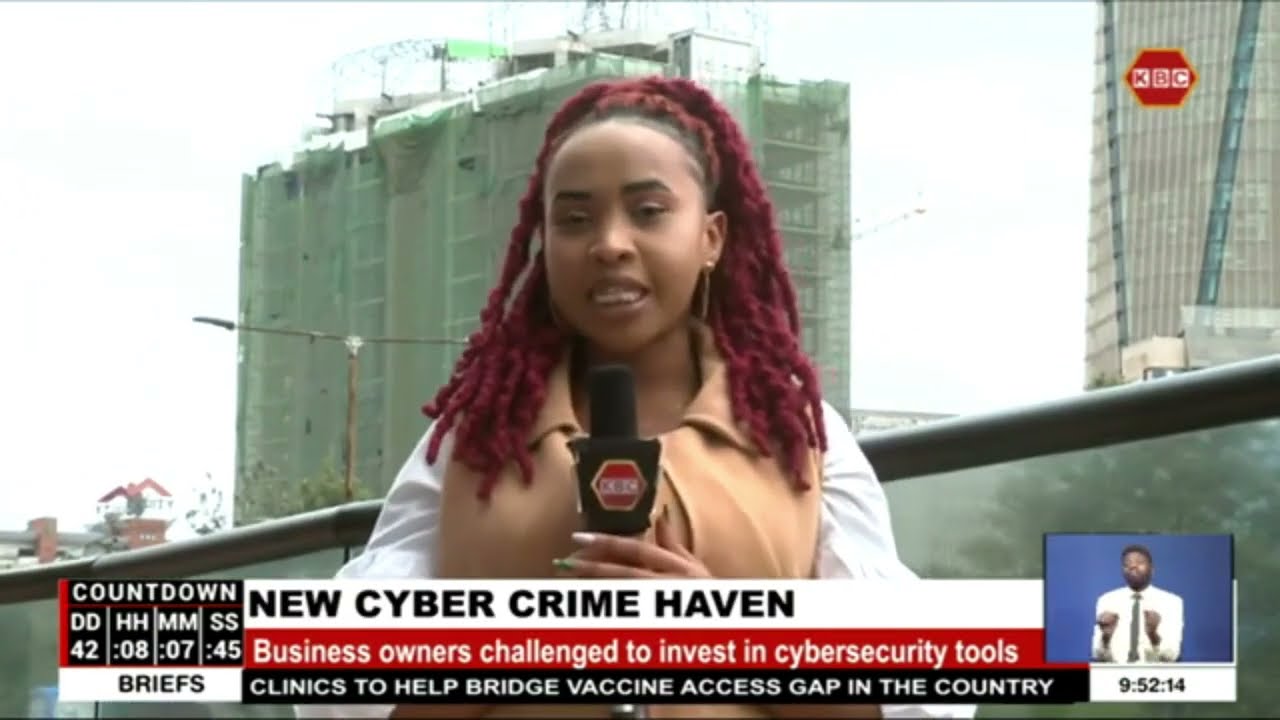The image is a photograph of a news telecast featuring a live outdoor report. The main focus is a black woman, likely the reporter, with distinctive long purple braids that resemble curly dreadlocks. She is wearing a peach or beige-colored sleeveless vest over a white shirt and is holding a black microphone marked with a red hexagonal logo bearing the letters “KBC.” Her dark eyes and eyebrows are prominent, and she wears earrings. Her mouth is open, likely speaking live.

In the background, there are tall buildings, possibly apartment blocks under construction, discernible by the scaffolding and a green tarp or mesh covering them. Behind her is a railing and a gray wall. The sky is overcast, appearing gray.

At the bottom of the image, several headlines and banners convey news topics: “New Cybercrime Haven,” “Business Owners Challenged to Invest in Cyber Security Tools,” and “Clinics to Help Bridge Vaccine Access Gap in the Country.” To the left, a countdown timer displays “42 days, 8 hours, 7 minutes, 45 seconds” with the word “Briefs” underneath, while on the right, a small inset shows a man on a blue background performing sign language, labeled with the time “9:52:14.” The news channel logo “KBC," in a red hexagon with white lettering, is situated in the top right corner.